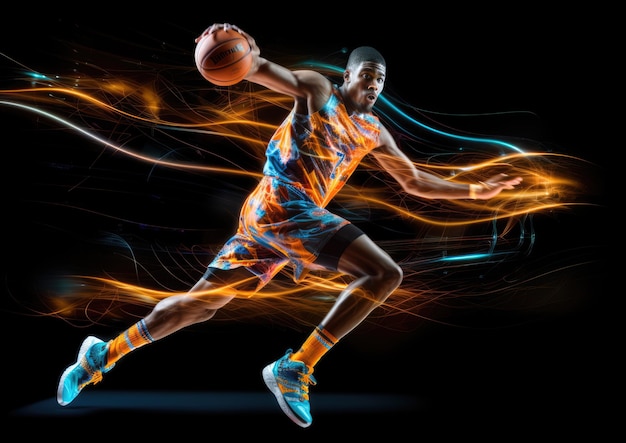This is a digitally altered poster depicting an African American basketball player mid-run, captured in a side view. The athlete, who appears tall and muscular with short dark hair, dons a vibrant uniform consisting of an orange and blue tank top and shorts with black borders. Coordinating with his outfit, he wears orange socks and blue sneakers with a white base. The player holds an orange basketball in his right hand, poised as if about to dribble, with his arms outstretched and mouth open in a focused expression. His head is slightly bent towards the viewer. Surrounding the player are dynamic orange and blue lines, enhanced through digital editing, which trail his movement. The background is predominantly black, except for a blue gradient near his shoes, adding depth and contrast to the composition.